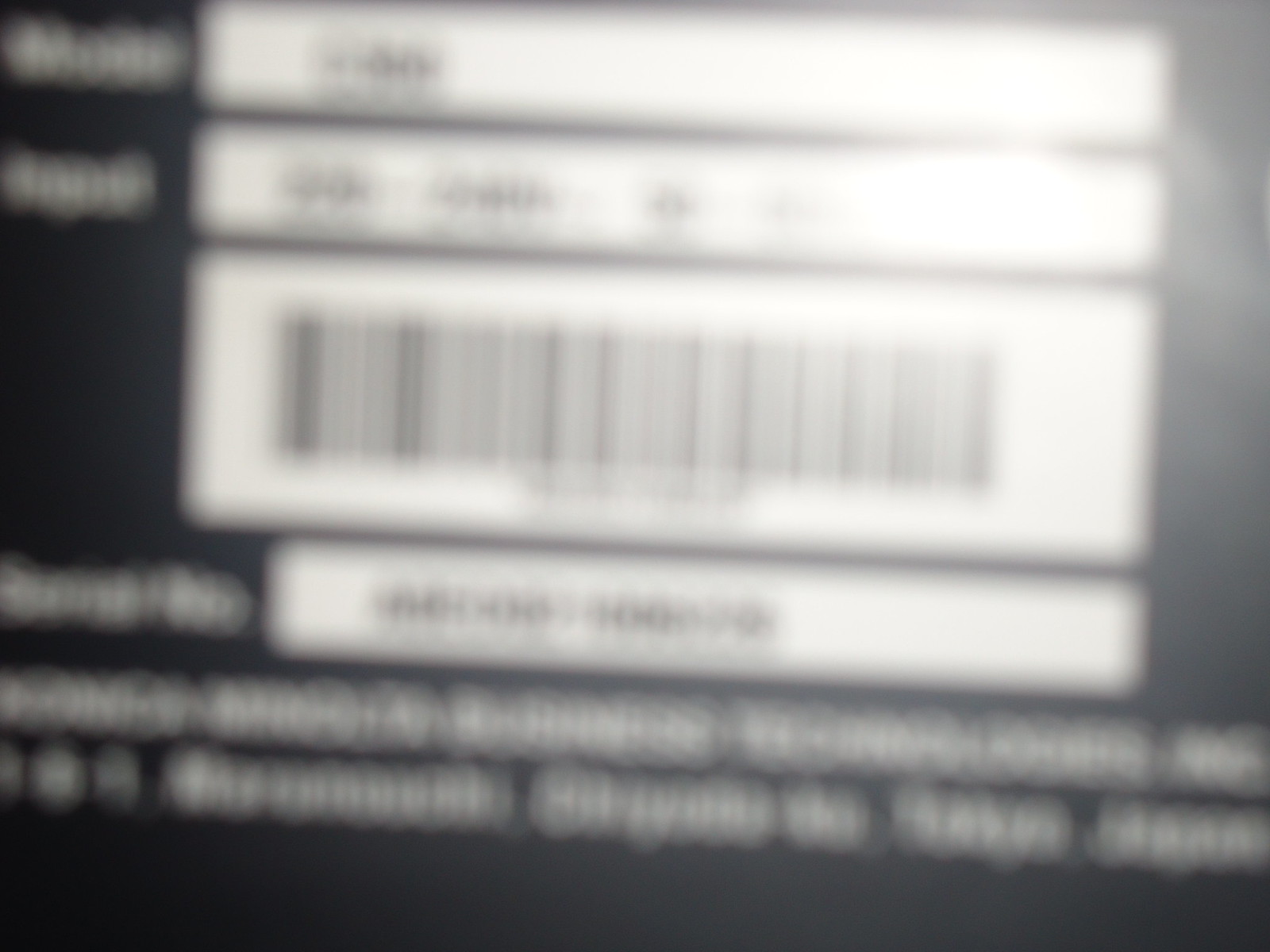The image features a blurry, landscape-oriented view of the back of an electronic device against a black background that fades lighter to the right. Prominently, four rectangular white strips with blurred black text are arranged in the middle, with the top strip containing the word "MODE" in white letters. Below this, a blurry UPC barcode is visible, followed by a sequence of numbers that become increasingly indistinguishable towards the bottom. Additionally, there is some barely legible larger white text located at the bottom of the image. The left side of the image is darker, while a brighter light illuminates the right side, creating a gradient effect.